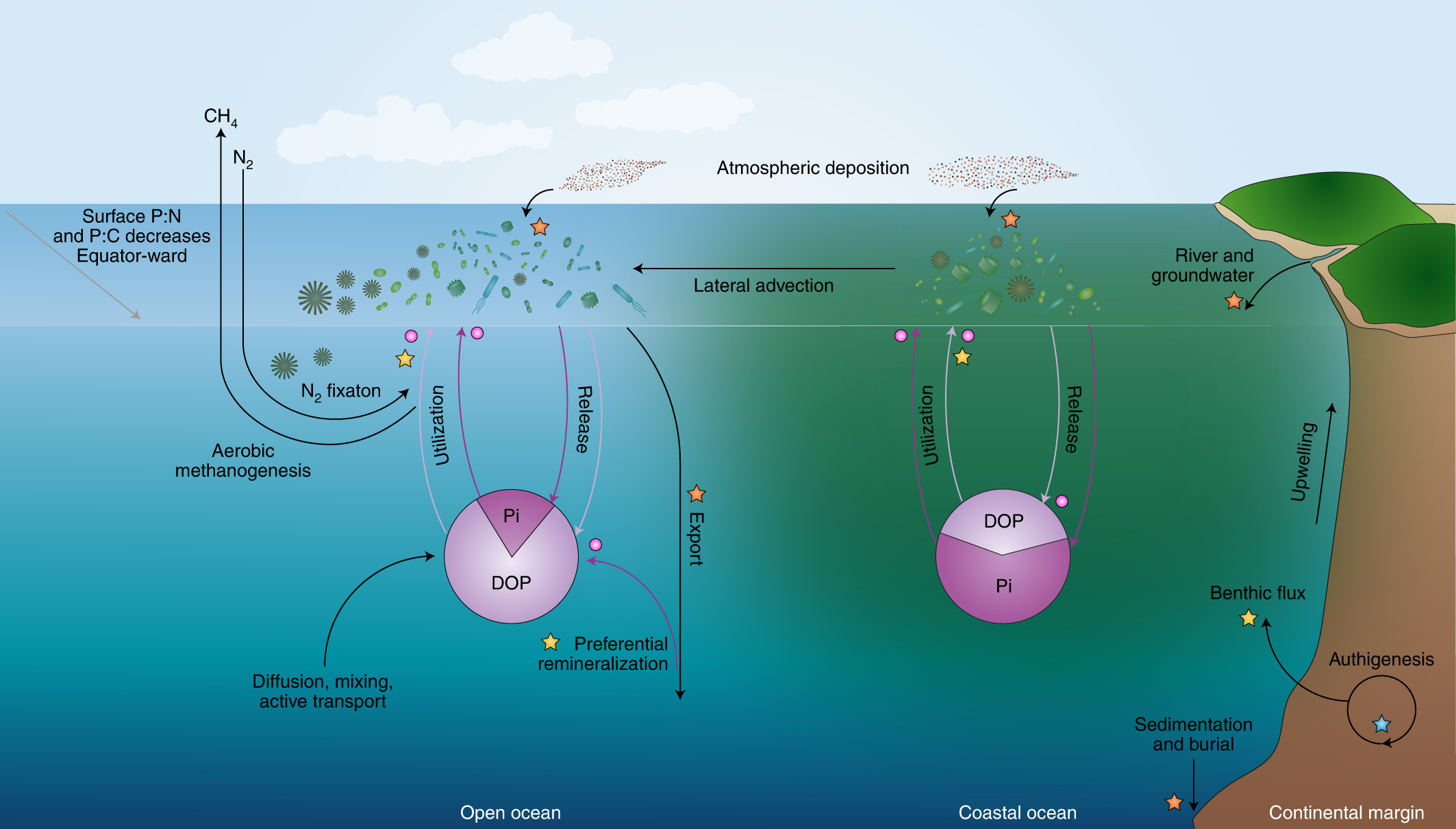The image is a detailed informational chart depicting the interaction and flow of elements between land and ocean. It features various lines of black text, images, and arrows, illustrating a large body of water, a coastal ocean, and a piece of land. The upper part of the image shows a blue area with lighter blue and white clouds, representing the atmosphere. Below this is a digital depiction of water, segmented into different processes.

Key components include the reduction of surface PN and PC as it moves equatorward, with detailed processes like CH4 and N2 production, N2 fixation, aerobic methanogenesis, utilization, release, diffusion, mixing, and active transport. The chart also mentions PI, DOP, open ocean, preferential remineralization, export, lateral advection, atmospheric deposition, and more.

On the right-hand side, a brown landform with grass and labels such as "continental margin" and "geothermal" is visible. Rain and groundwater runoff into this water body, showing labels for upwelling, sedimentation, and burial, including terms like orthogenesis and benthic flux.

Overall, the chart illustrates the comprehensive cycle and interaction of matter from river and groundwater through processes like upwelling, benthic flux, continental margin interaction, sedimentation, burial, and various chemical and biological transformations spanning the coastal and open ocean environments.